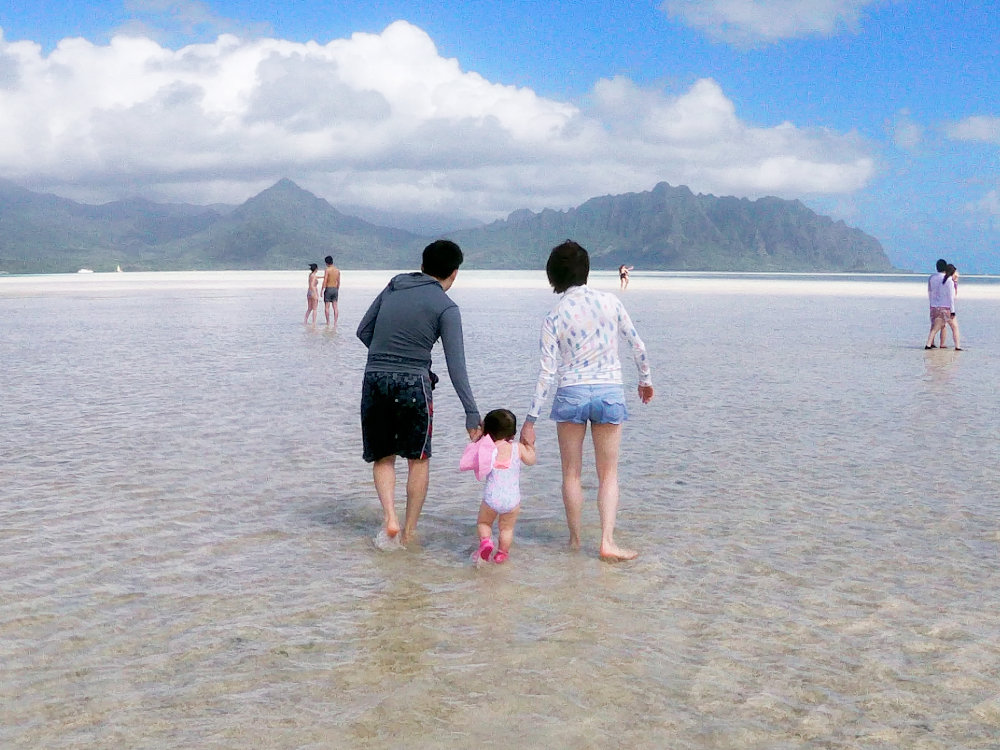This is a large, square, grainy picture of a family at a beach, with the upper part dominated by a clear blue sky filled with large white clouds that have gray bottoms, especially on the left side and in the middle. In the center background, a mountain range appears as a greenish outline under the sky. The water is very shallow, barely covering the feet of the people wading through it, so the brown sand underneath is visible. 

In the foreground, seen from behind, a man and a woman are each holding the hands of a small child, who is walking between them. The child is wearing pink shoes and a white swimsuit. The man is dressed in a long sleeve dark gray hooded shirt and black swim trunks, and is barefoot. The woman is also barefoot, wearing very short cut-off denim shorts and a patterned white long sleeve shirt. Both adults have short black hair, and all appear to be Asian, suggesting the setting might be in an Asian country.

To the right, in the distance, another pair of people can be seen embracing. On the left side, a couple is also visible, and far out towards the horizon, there appears to be a sailboat. The beach and shallow waters extend into the background, with more groups of people scattered throughout the scene.